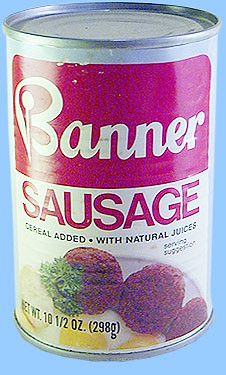This vintage photograph captures an old advertisement for a canned food product called Banner Sausage, indicative of its age through the faded colors and magazine-like quality. The label of the can is prominently featured, divided into distinct sections. At the top, a striking red rectangle displays the brand name "Banner" in an elegant cursive white font. Directly beneath, "Sausage" is written in bold red capital letters against a clean white background, drawing immediate attention. Further details on the label include the phrases "Cereal Added with Natural Juices" and "Serving Suggestion," providing potential cooking ideas for consumers. An appetizing serving suggestion is depicted in the photograph: a plate showcasing three sausages accompanied by a fried egg and unidentified side, garnished with fresh parsley. The background of the product image is a solid blue, contrasting with the elements on the label to create a visually appealing presentation.